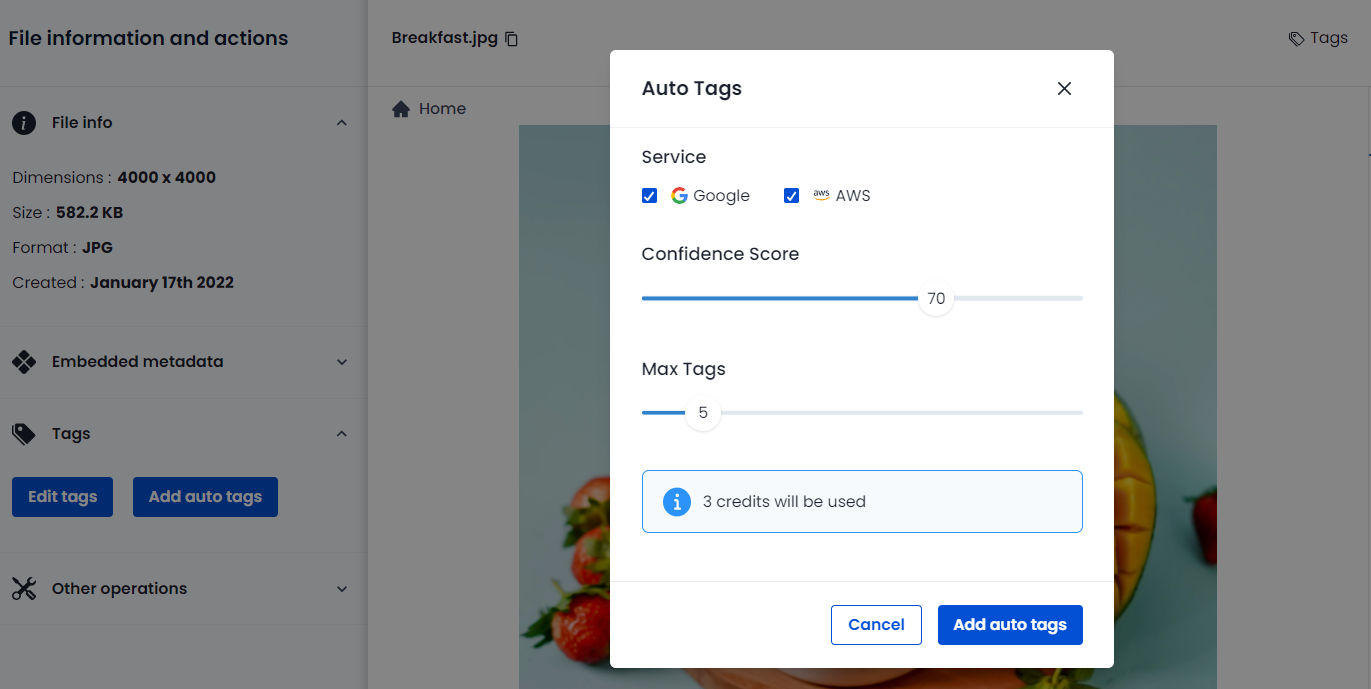The image features a grey background with a grey rectangle prominently displayed. On the left side of the rectangle, there is a section titled "File Information and Actions." A black circle with an illustrated eye icon is present nearby, accompanied by text and numbers in grey and black hues.

Below that, a sequence of text lines follows, each consisting of grey and black words and numbers. One line specifically includes a date displayed in black. Further down, a diamond shape composed of smaller diamonds is visible, with adjacent text and a downward-pointing arrow. There is also an icon resembling a tag with accompanying text and an upward-pointing arrow.

Toward the bottom, two blue rectangles are labeled "Edit Tags" and "Add Auto Tags." A section titled "Other Operations" with an adjacent downward-pointing arrow is also present.

On the top left corner, there's a file name displayed, while on the right side, a symbol and the word "Tags" are visible. An icon depicting a house is labeled "Home." 

The majority of the background picture is obscured by a superimposed white rectangle that reads "Auto Tags" on the left, with an "X" for closing on the right. This section also includes the term "Service," with a blue square featuring a check mark next to the Google "G" logo labeled "Google." Similarly, another blue square with a check mark is next to a symbol labeled "AWS."

Additional indicators include a "Confidence Score" with a blue progress line extending to 70, then continuing as a grey line. For "Max Tags," there is a blue line reaching the number 5, followed by a grey line. Lastly, a blue rectangle contains a blue circle with a light blue eye icon, under which it notes, "Three credits will be used."

At the bottom of the section, a blue-outlined rectangle labeled "Cancel" and a blue rectangle labeled "Add Auto Tags" are present.